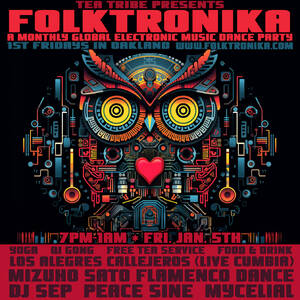This captivating poster features a dark black background, in the center of which stands an intricately designed mechanical owl, composed of various electronic and metallic components. The owl's eyes are striking yellow circles, with red and black feather-like eyebrows, and its beak forms a red heart shape. The owl is rendered in shades of grey, blue, yellow, and orange, creating a vivid and colorful central image.

At the top of the poster, bold red text announces "T-Tribe Presents," followed by the main event title "FOLKTRONICA" in large, all-capital letters in an even brighter shade of red. The poster reveals that Folktronica is a monthly global electronic music dance party. Beneath this, in blue text, it adds further information: "First Fridays in Oakland, www.folktronica.com."

Below the owl, details of the event are provided: the party is scheduled for 7 pm to 1 am on Friday, January 5th. The red background beneath contains a list of performers including Yoga, DJ Gong, Free Tea Service, Food and Drink, Los Alegres, Calejandros, and Vivecambia, with additional text in Spanish. The overall design combines vibrant colors and mechanical elements to create an eye-catching and unique promotional image.